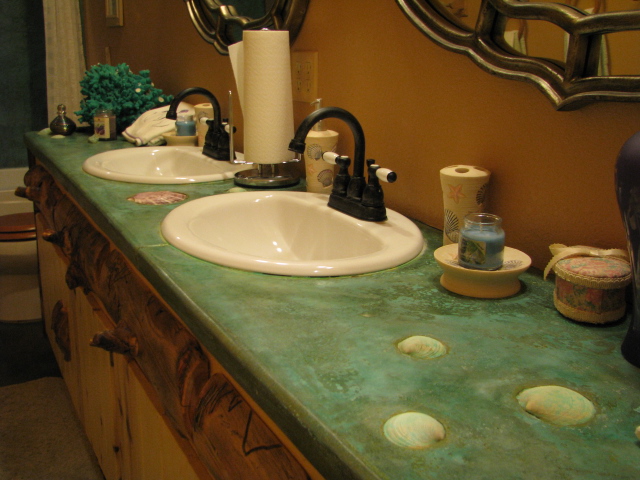A beautifully designed bathroom featuring a long, marbled countertop in varying shades of green and dark green, extending the full length of the burnt orange-colored wall. Large, ornate mirrors with gold accents are affixed to the wall, wonderfully reflecting light. Embedded within the countertop are three large white seashells, speckled with hints of green, and a single pinkish shell positioned centrally between two pristine white sinks. The sinks are complemented by bronzed faucets with elegant white handles. To the left, a white toothbrush holder decorated with miniature seashells is neatly placed. A small dish containing a blue candle sits nearby, adding a touch of tranquility to the space. Toward the back, close to the toilet, a lush green plant provides a refreshing burst of greenery. The front of the cabinets showcases a decorative wood-like finish, enhancing the overall warmth and charm of the bathroom.